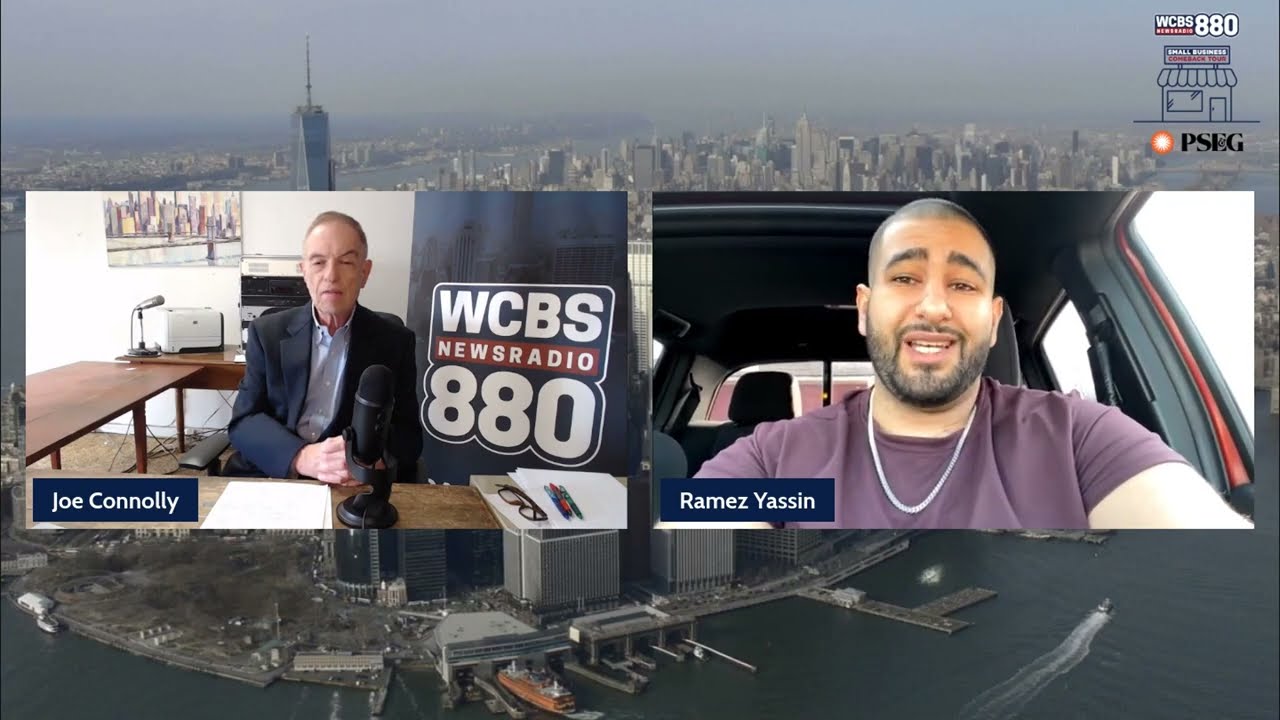The image depicts a split-screen radio news interview between two individuals with a detailed city skyline and a foggy sky in the background. On the left side, Joe Connolly, an older man with a black suit and light blue undershirt, is seen seated at a desk with a radio microphone in front of him. Additional items on his desk include a cup, a white piece of paper, pens, and glasses, while behind him, there are posters, a light, a printer, and various objects. The setting clearly indicates he is inside a recording studio with the WCBS Newsradio 880 logo prominently displayed.

To the right side of the screen, Ramesh Yassin, a younger man with a beard and a neatly outlined mustache connecting to a dark chin beard, appears to be inside a car, evidenced by the visible back seats and seatbelt. He is wearing a purple shirt with a white necklace. The bottom portion of the image shows a drawing featuring a small house with a window and door, a sun symbol, and the PSEG logo. An aerial photograph of a city skyline, possibly Chicago, with tall skyscrapers, further enhances the background setting. The overlay identifiers in the image affirm the names of the host and guest as Joe Connolly and Ramesh Yassin, respectively.